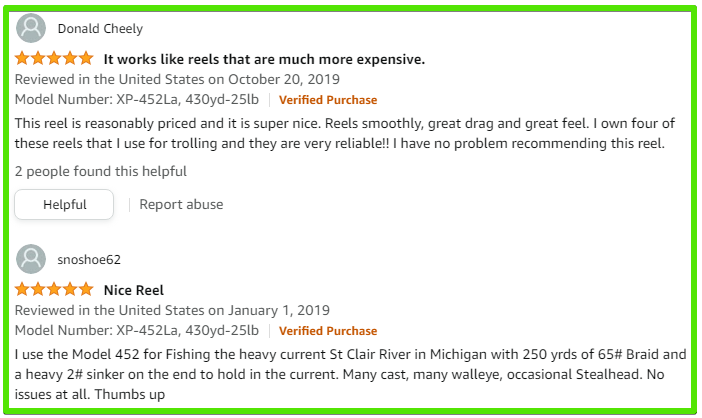The image features a white box with a green border. Inside the box is a generic profile picture alongside the name "Donald Cheely," who rated the product 5 stars. In bold text, the caption states, "It works like reels that are much more expensive." Below this, in gray text, it notes, "Reviewed in the United States on October 20th, 2019." The bottle number "XP-452LA430YD-25LB" and "Verified Purchase" are also mentioned.

The review further elaborates that the reel is reasonably priced yet exceptionally nice, mentioning its smooth operation, great drag, and excellent feel. Donald Cheely states he owns four of these reels for trolling and finds them very reliable, confidently recommending them to others. 

Additionally, it indicates that "Two people found this helpful." 

Below this review, another similar review is summarized with the highlighted notes: "No Shoes 62" has also rated the reel 5 stars, calling it a "nice reel" and noting that their review was posted on January 1st, 2019, with the same bottle number "XP-452LA430YD-25LB" and "Verified Purchase" label.